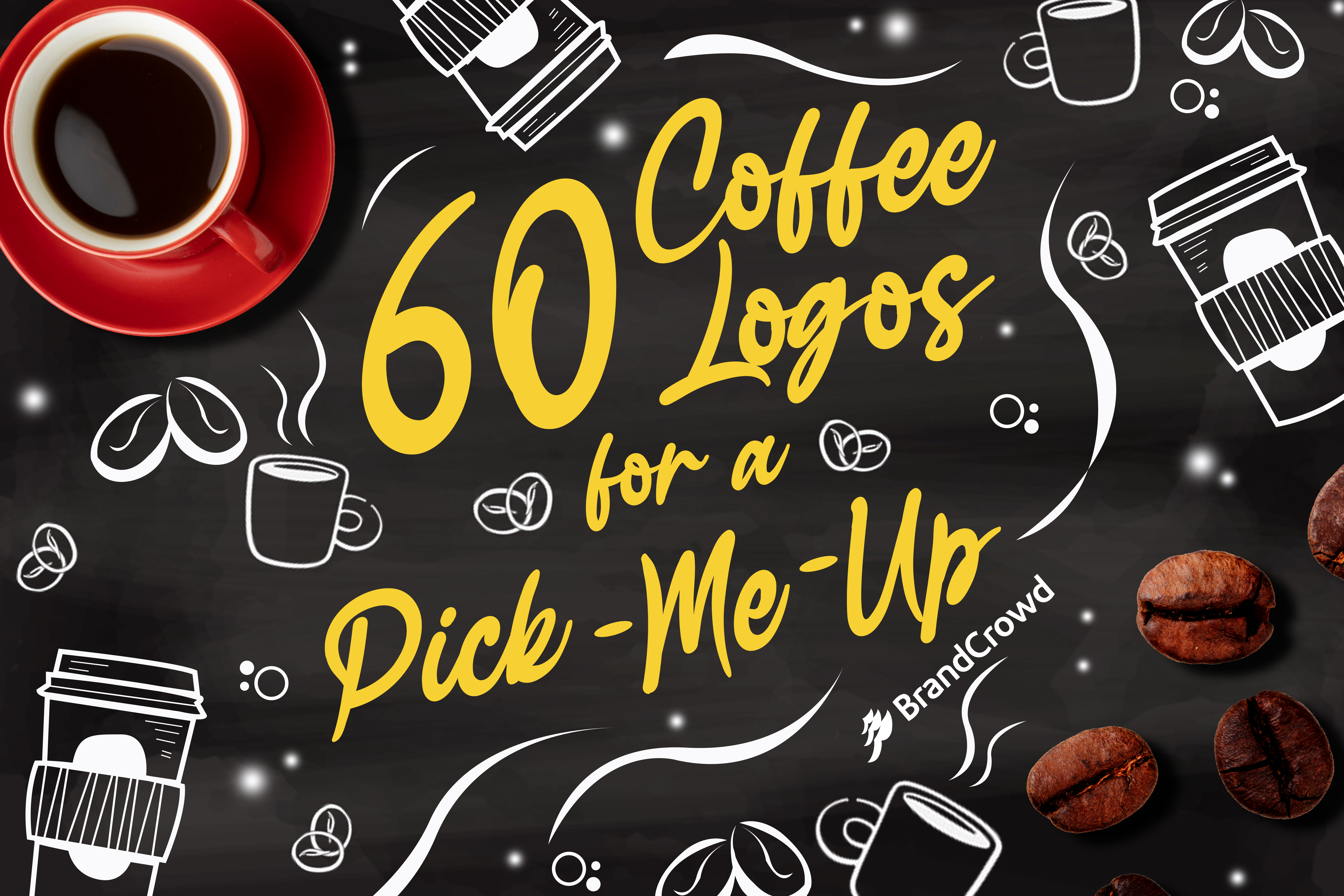This image advertisement for a coffee shop or coffee brand called Brand Crowd features a meticulously crafted chalkboard-style design. At the heart of this computer rendition, designed to mimic a black chalkboard, are large, bright yellow calligraphy-style letters that announce "60 Coffee Logos for a Pick-Me-Up." Surrounding this central text are artistically rendered decorations—chalk-like illustrations of to-go coffee cups, steaming coffee mugs, and scattered coffee beans, all contributing to a cozy, handcrafted feel. The brand name "Brand Crowd" is subtly written in smaller white letters. Enhancing the visual appeal, a vibrant red coffee mug filled with black coffee sits in the top left corner, while freshly roasted coffee beans are displayed in the bottom right, adding a touch of realism to the chalkboard aesthetic. Swirling lines interlace the design, further enriching the dynamic, inviting atmosphere of this coffee lovers' haven.